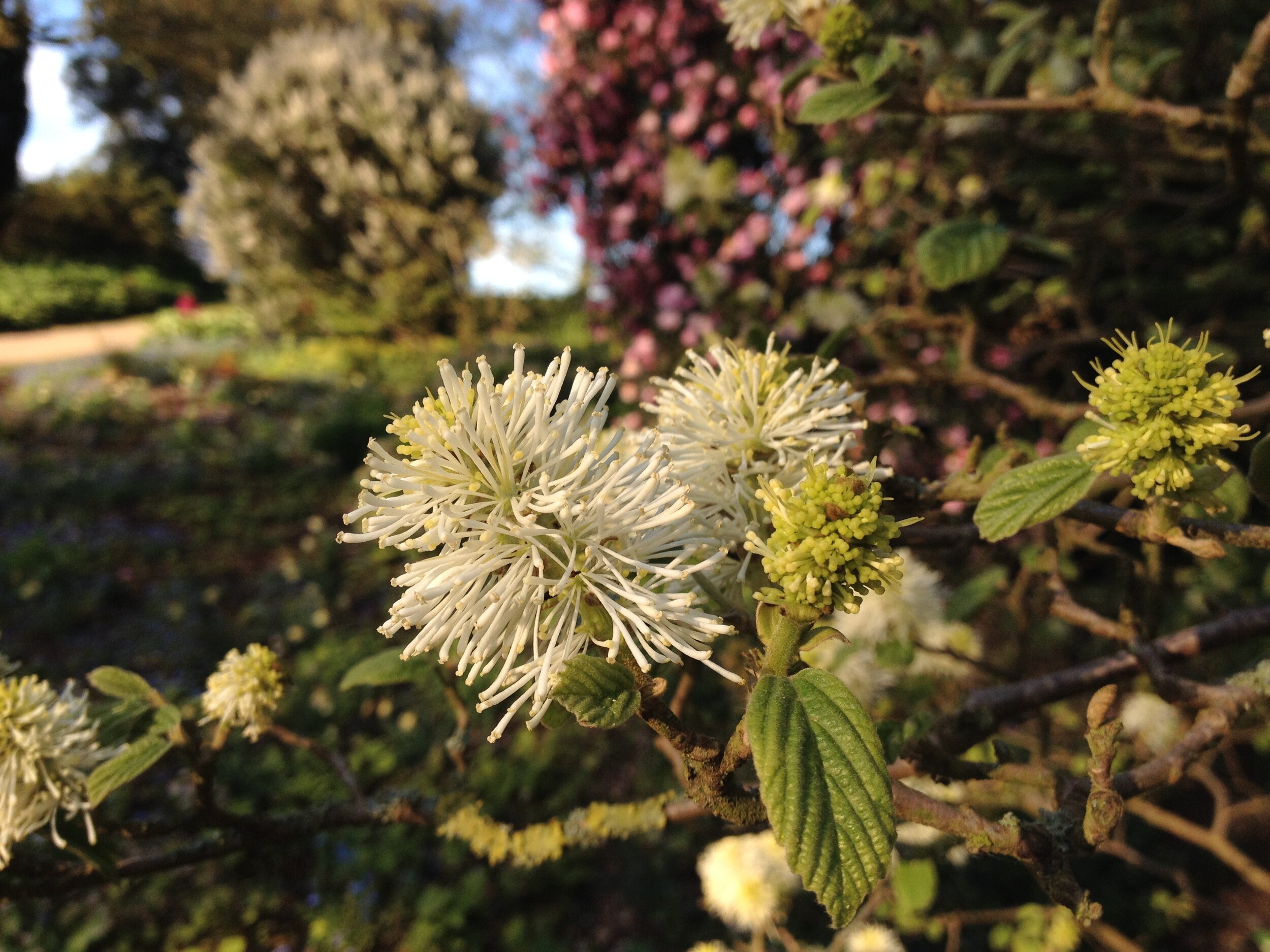The photograph, likely taken with a high-quality camera, captures a detailed close-up of a large white flower in bloom amid a picturesque garden scene. The flower, adorned with a multitude of soft, tentacle-like petals and prominent yellow pollen, stands prominently in the middle of the frame, attached to green leaves and accompanied by a nearby bud yet to bloom. In the blurred background, a diverse and lush landscape unfolds. Blooming trees, shrubs, and flowers populate the scene, including a flowering bush with white blossoms and another with pink, possibly an azalea. The scene unfolds on a sunny spring day, with a glimpse of a green yard, a path or driveway in the upper left, and a stretch of clear blue sky, all contributing to the tranquil beauty of nature in its full bloom.